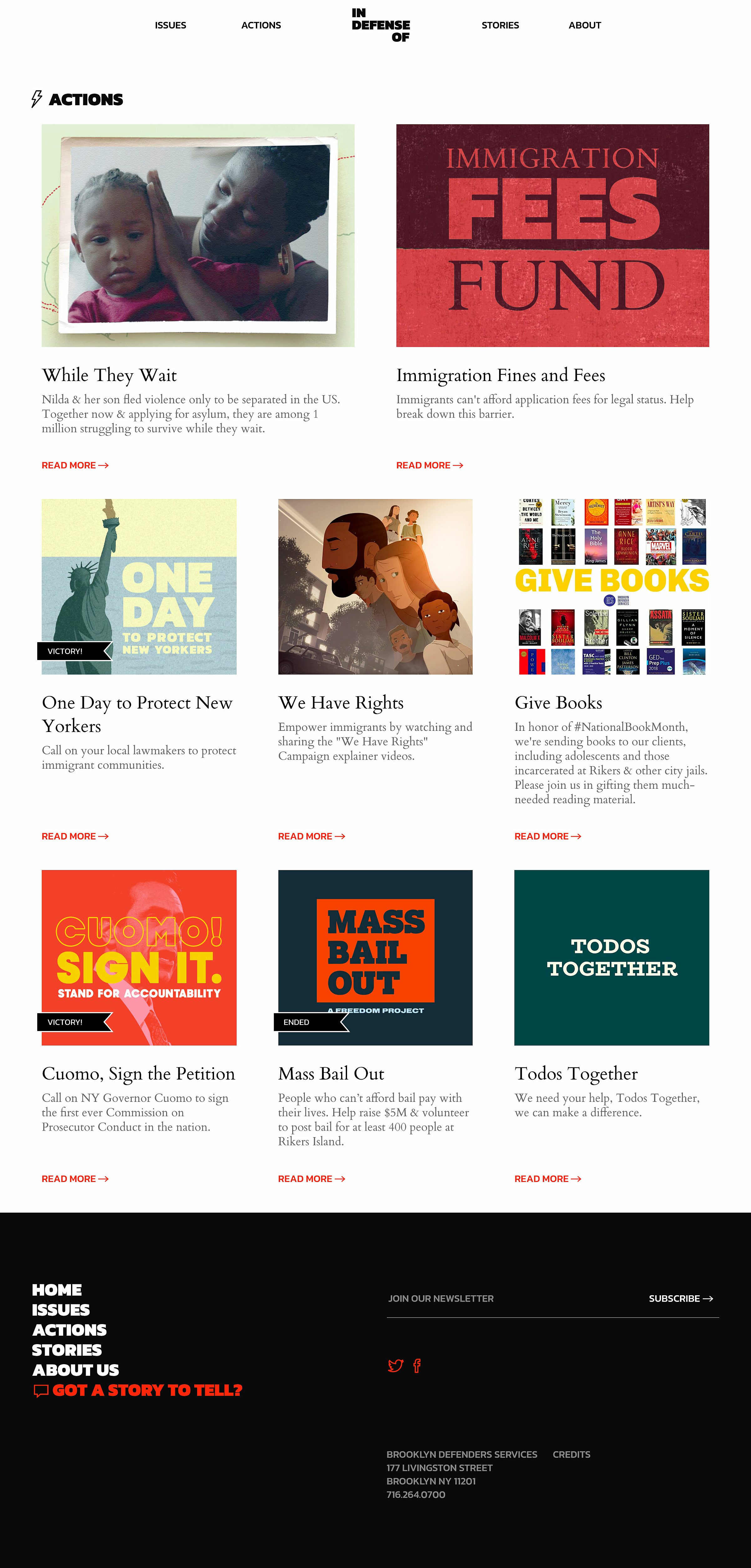This is a website with a rather confusing layout. At the top, there is a date range spanning five days, though the purpose of this information is not immediately clear. The main section below houses several action-oriented sections, seemingly aimed at various social causes. There are eight clickable images, each representing a different page titled "Actions."

1. The first section is titled “Why They Wait” and features an image of an African American mother and her child.
2. The next section is labeled “Immigration Fees Fund,” presented in block letters with shades of off-red and dark maroon.
3. “One Day to Protect New Yorkers” is accompanied by an image of the Statue of Liberty.
4. Another section, “We Have Rights,” features a drawing of a man, a woman, and a child.
5. “Give Books” is illustrated by a small picture of a collection of books.

The remaining three sections were not described in detail, but they likely have similar action-oriented themes. The overall presentation is somewhat disorganized, making it challenging to grasp the website's full purpose at a glance.